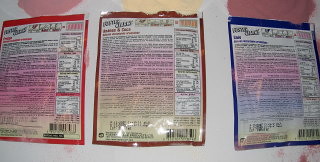This photograph features a trio of product bags displayed side-by-side. The bag on the left stands out with a red outline, a white background, and black text, prominently featuring a gradient red design at its center. In the middle, the bag boasts a brown or orange outline, a white background, black text, and a captivating gradient shifting from pink to orange. The rightmost bag is distinguished by its blue outline, a white background, black text, and a stunning gradient that transitions from pink to blue. Each bag is marked with a barcode in the bottom right corner and has an ingredient label on its right side. The items are arranged on a surface that resembles a Twister mat, adding a playful and colorful backdrop to the display.